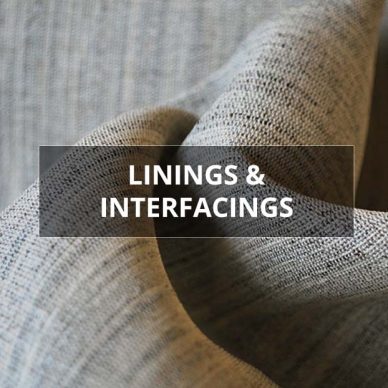The image is a close-up square photograph of patterned fabric, featuring vertical strips in a blended light brown, dark brown, and beige color palette. The upper left portion of the image appears blurry, emphasizing the intricate pattern of the fabric. The right side and bottom left portion show the fabric rolled up and folded over. Dominating the center of the image is a dark gray rectangle outlined in white, overlaid on top of the fabric. Inside this rectangle, the words "LININGS AND INTERFACINGS" are prominently displayed in all-uppercase white letters. The picture is well-lit, likely due to natural daylight or a flash, and is devoid of any other text, numbers, or people.